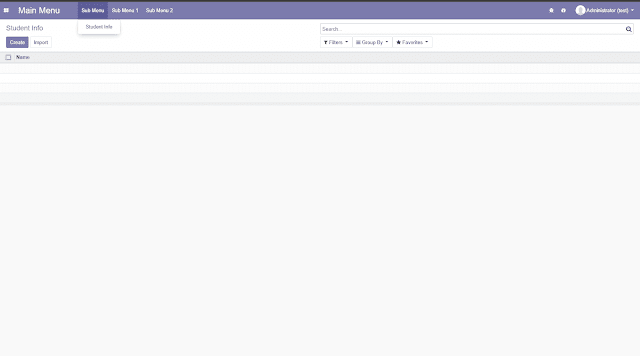A screenshot of an open application on a desktop computer displays various interface elements. At the very top, a purple banner features white text reading "Main Menu," followed by "Submenu," "Submenu 1," and "Submenu 2." On the far right of the banner, there is an "Administrator" label next to a white circle containing a black silhouette of a person. Below the banner, a white bar presents options such as "Student Info," "Student File," and "Import," along with a search field characterized by a black magnifying glass icon. Further down, drop-down menus labeled "Filters," "Group By," and "Favorite" are aligned horizontally. Below these, a gray rectangle contains a black checkbox labeled "Names." The section beneath this has three white rectangles, followed by another gray rectangle, leading to a large empty grey area, indicating an unused or empty menu space.